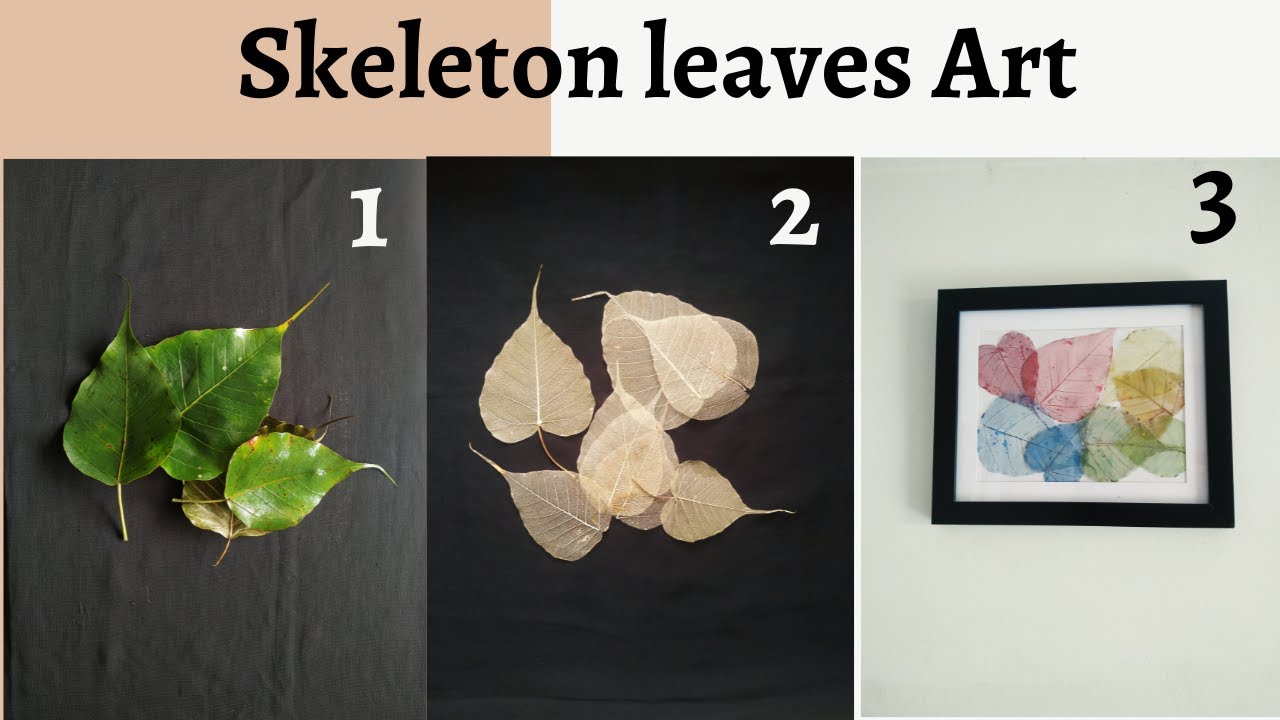The image displays a detailed progression of creating Skeleton Leaves Art. At the top, a two-toned border—light brown transitioning to white—hosts the title in bold black letters: "Skeleton Leaves Art." The artwork's transformation unfolds in three labeled panels below this header.

Panel 1, set against a dark gray background, features three small green leaves, freshly picked and intact. In Panel 2, the backdrop turns black, highlighting around ten heart-shaped leaves that have lost their green pigment, appearing now in a translucent, pale tan color. Panel 3 completes the transformation, showing these same leaves vibrantly dyed in pastel hues of pink, blue, red, yellow, and green. These colorful leaves are arranged as wall art within a black frame, bordered in white, and displayed on a pale green wall. This visually striking sequence demonstrates the intricate evolution from natural green leaves to their final, creatively colored state.